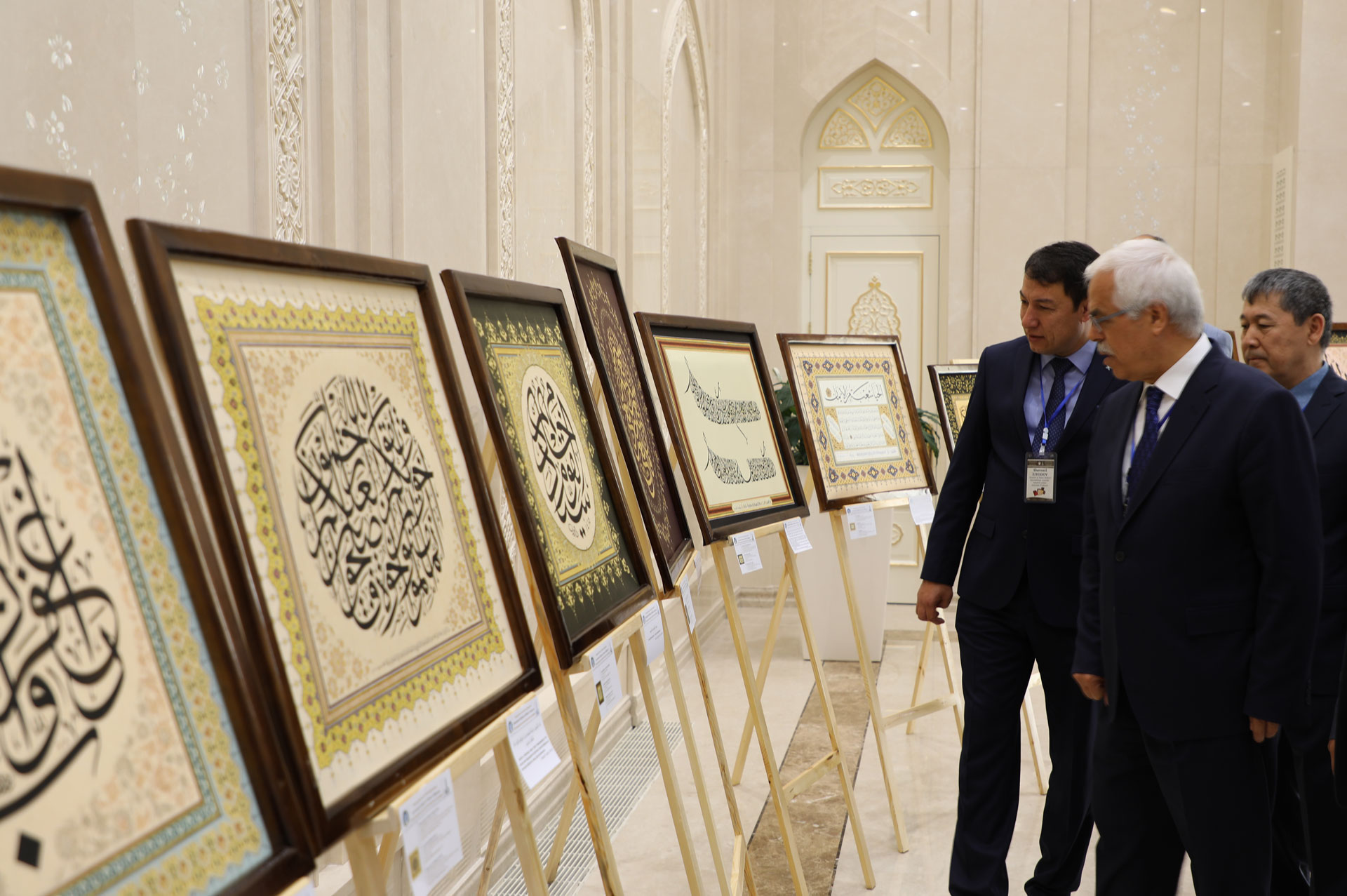This color photograph, taken indoors, captures a gallery setting with three men on the right-hand side, all dressed in dark suits. One man, with gray hair and glasses, stands slightly ahead of the others, who are wearing blue shirts and dark ties — one of them also has a lanyard around his neck. They are intently observing a row of seven framed pieces on wooden easels, each frame brown and containing detailed, rounded designs that appear to be ornate calligraphy or intricate drawings. Each framed piece has a decorative label at the bottom, suggesting an exhibit or museum setting. The room has light beige or sandstone-colored marble floors and walls, enhancing the elegance of the display environment.